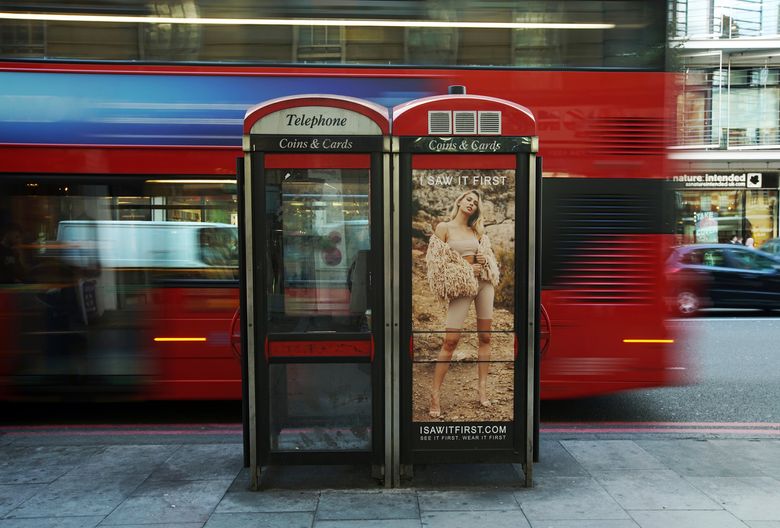The image captures two distinctive black phone booths with red, domed roofs, set on a gray-tiled city street in London, England. The phone booth on the left prominently features the word "Telephone" in black, with a lower bar reading "Coins and Cards" in white lettering against a black background. The right phone booth showcases an advertisement for a fashion website, I Saw It First. The ad displays a young woman modeling a light tan fur ensemble, including leggings and a bra top, standing against a dirt hillside.

In the blurred background, evidence of a long-exposure shot, a red double-decker bus is visible, moving from the right to the left side of the image. The bus features a blue advertisement separating its upper and lower decks, accentuating its iconic London appearance. Behind the bus, blurred outlines of other cars and various buildings, potentially apartments or stores, occupy the cityscape. The image vividly captures the bustling energy of London, with its blurred transportation and iconic elements.